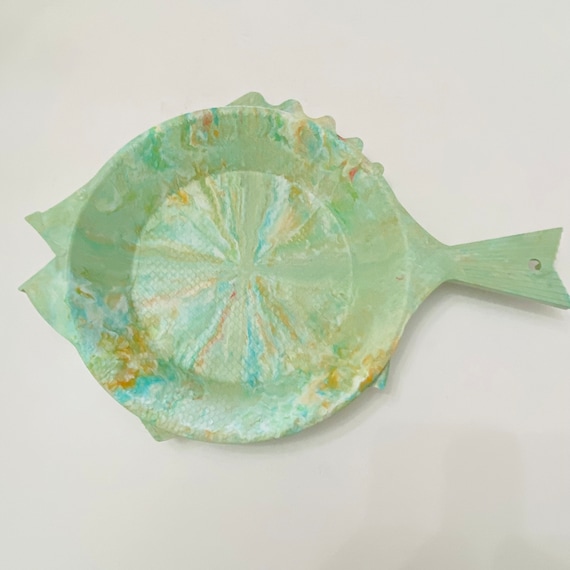The image features a ceramic or marble dish, meticulously crafted to resemble a fish. The dish is set against a gray background and showcases a unique design with intricate details and a plethora of colors. The base of the dish is circular, rising up into a shallow bowl. The left edge of this bowl extends into two triangular points, mimicking fish lips, while the upper edge has a ripple-like feature stretching from the center to the right side, representing a fin.

Further enhancing its aquatic theme, the right side of the dish flares into a triangular shape with engraved fan-like textures, resembling a fish tail. This tail acts as a practical handle for the plate. The entire piece is adorned with swirls of orange, cream, turquoise, light green, and darker green hues, which radiate from the center, creating a dynamic and vivid visual effect. Blue and brownish tones are also present, adding to the dish's depth and complexity. An eye is distinctly visible on the upper left part, completing the fish motif. The dish appears to be molded as one cohesive piece, possibly crafted from clay or ceramics, with fine attention to detail that suggests it could be used as a serving dish, coaster, or even an artistic ashtray. A light source illuminates the left side of the image, highlighting the dish's textured surface and vibrant colors.